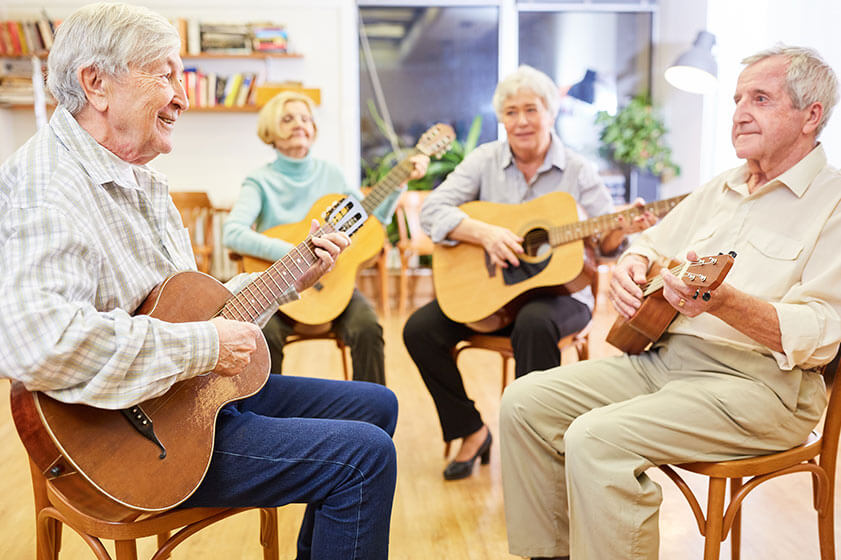In a cozy indoor setting, four elderly individuals, all appearing to be in their late 70s to early 80s, are seated on wooden chairs, deeply engaged in playing guitars. The scene is illuminated by a blue lamp with a white bulb, casting a warm glow over the room. A white wall and a sliding glass door form the backdrop, adding a touch of serene simplicity, while shelves brimming with books and lush green plants create an inviting ambiance.

All four musicians have gray hair and are casually dressed in long-sleeved, button-up shirts. The men, dressed respectively in a white and beige checkered shirt with blue jeans and a beige shirt with beige pants, sit opposite each other in the foreground. The man in the checkered shirt cradles a brown, well-worn guitar characterized by scratch marks below the opening, indicating years of use. The man in khakis appears to be playing a smaller string instrument, possibly a ukulele.

Behind them, the two women are also seated, contributing to the harmonious guitar ensemble. One woman, adorned in a blue sweater, has short blonde hair and is wearing green pants, while the other, with short grey hair, sports a blue button-down shirt, black pants, and black heels. Their guitars vary in color and style, with the woman in the blue sweater holding a lighter-colored guitar.

The group seems united in their musical endeavor, their attention collectively focused on the man in the white and beige checkered shirt, who appears to be leading the session. This snapshot captures not only a moment of musical collaboration but also an intimate glimpse into the joy and camaraderie shared among these seasoned musicians.